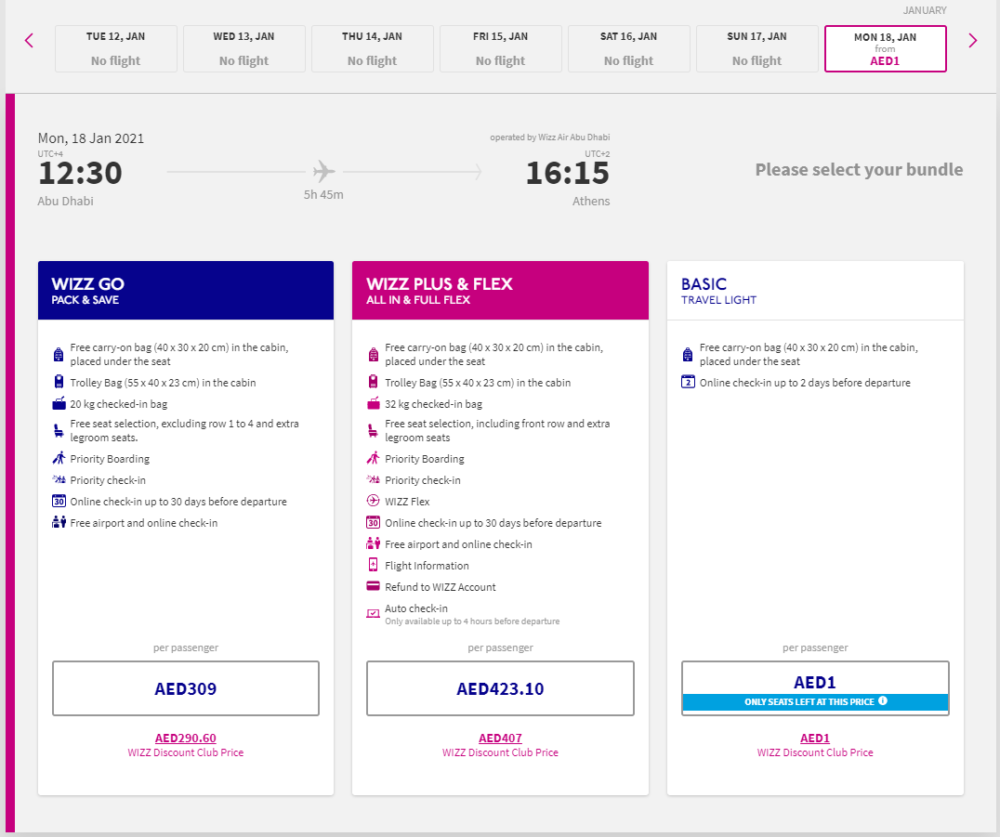This vertical image, which could be encountered on a website or a smart device, features a medium gray background. Positioned in the upper left corner, a mauve arrow points downward and to the left. To the right of this arrow, a header elaborates on flight details in black bold text, followed by availability information in gray.

The text details flight availability from Tuesday, January 12th to Sunday, January 17th, indicating no flights on each of those days. However, on Monday, January 18th, a flight is available, starting from AED 1, highlighted within a box.

Detailed flight information for January 18th, 2021, is given:
- Departure: 12:30 PM from Abu Dhabi
- Duration: 5 hours and 45 minutes
- Arrival: 16:15 (Military Time) in Athens
- Instruction: "Please select your bundle"

Three bundles are offered:
1. **Wizz & Go and Pack & Save** (Blue strip): Details for each option are included within the respective sections.
2. **Wizz Plus and Flex** (Mauve strip): Descriptions for each choice are laid out, marked under subheadings "All In" and "Flex."
3. **Basic Travel Light**: Allows for a selection of a minimalistic travel option.

Users are invited to choose their preferred travel package from the presented options.